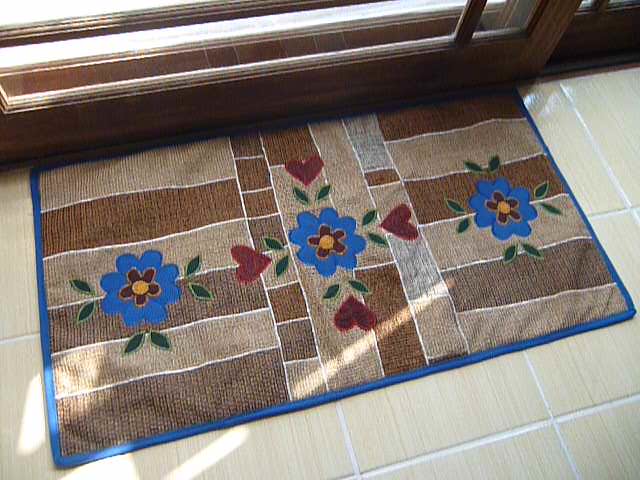This square-shaped, color photograph captures a detailed view of an indoor welcome mat, positioned on a light yellow or beige tiled floor. The mat, likely placed in front of a door with glass panes, features a prominent light blue border. The intricate design on the mat is composed of light brown and dark brown rectangular patterns with white lines between them. At the center of the mat, three striking blue flowers are aligned horizontally. Each flower, adorned with either red or yellow centers, is encircled by green leaves. The central flower is uniquely flanked by four red hearts and additional red leaf designs. Natural light streaming in from the window enhances the overall warmth and coziness of the scene.